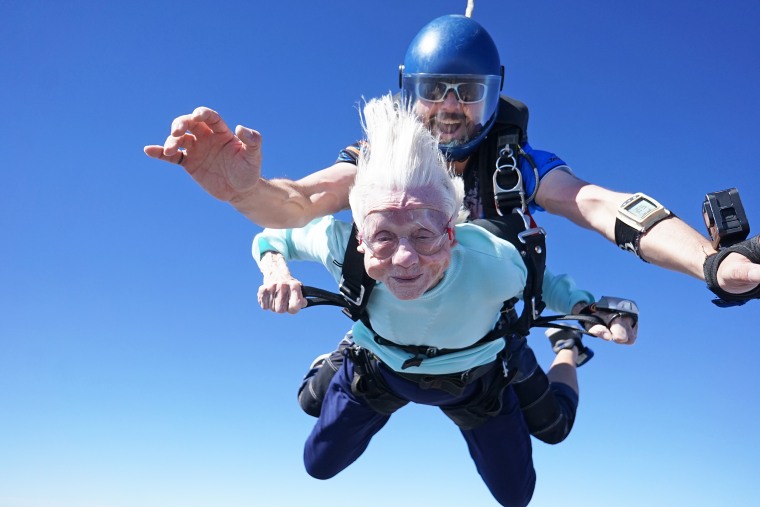This striking color photograph captures an exhilarating moment during a tandem skydiving experience against a backdrop of a clear, cloudless blue sky. Dominating the image is an elderly woman, possibly in her seventies or eighties, with her white hair streaming upwards and her wrinkled face being pulled back by the onrushing wind, reflecting both the excitement and the tension of the jump. She is not wearing goggles, which makes the distortion on her face more noticeable. Dressed in a light blue long-sleeved shirt and darker blue pants, she is securely strapped to her instructor. The black harness securing her to the instructor is clearly visible. 

Above and slightly behind her is the instructor, a man wearing a blue short-sleeved shirt and a dark blue helmet, which features a clear face visor. He also sports silver sunglasses, a beard, and is smiling confidently towards the camera. On his left arm, he has an instrument, possibly a watch or altimeter, strapped around his forearm and a GoPro mounted on a glove on his left hand, capturing footage of their adventure. His right arm is bare except for a ring on his pinky finger. Despite the thrill and chaos of the fall, he maintains a composed demeanor, in stark contrast to the concerned expression of the elderly woman below him. This vibrant image perfectly encapsulates the thrill and dynamics of skydiving, highlighting the bond of trust in a tandem jump amidst the vast expanse of the sky.